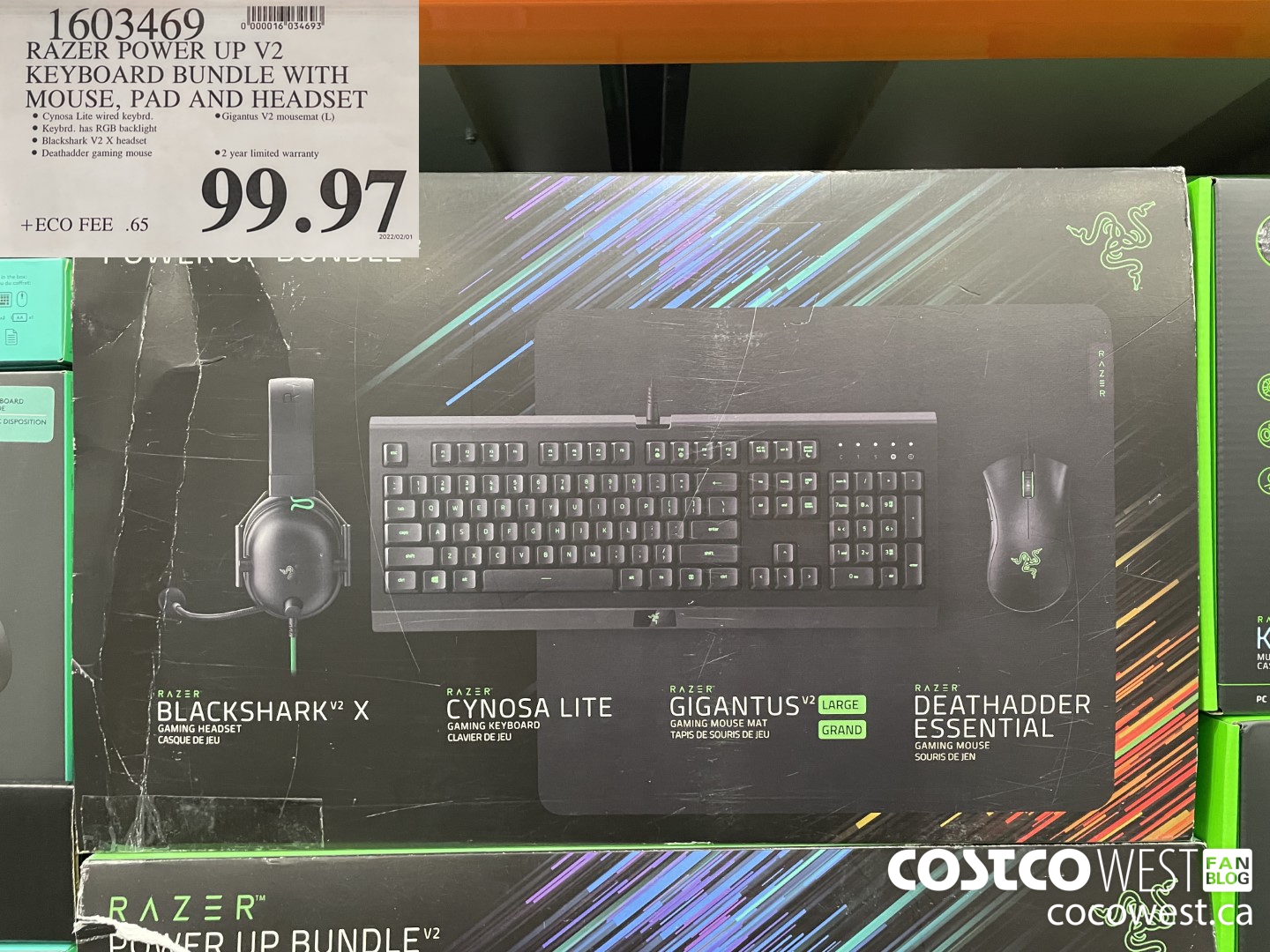The image depicts a store shelf with an orange-tinted edge, partially visible at the top. In the upper left corner, there's a piece of paper displaying a product label with various details. The paper lists items included in the bundle: "Razor Power Up," "Fee 2," and "Keyboard Bundle with Mouse Pad and Headset," along with different properties and a price of $9.97.

The product box appears to be slightly damaged, possibly due to shipping or a prior return, and is taped in the lower left corner. The box features images of a headset, a smartphone attached to one side of the headset, a wired keyboard, and a mouse. Specific product details on the box include a Razer BlackShark X gaming headset, Ksonar Lite gaming keyboard, Conegus large gaming mouse pad, and a Razer DeathAdder Essential gaming mouse.

In the lower right section of the image, "Costco West Fan Blog" and "CostcoWest.ca" are visible, indicating the store or fan blog associated with the image.